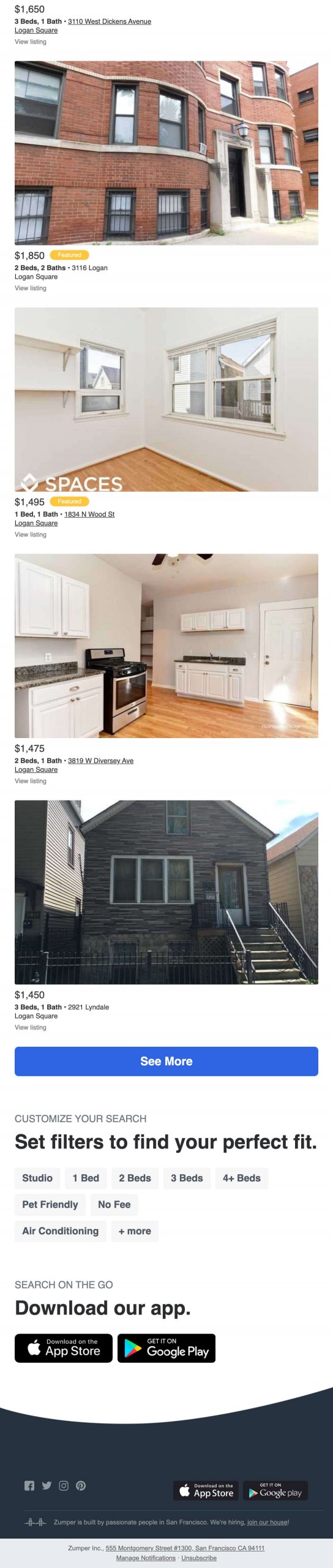Screenshot of a Property Listings Page: The image is a screenshot from an app or website showcasing various property listings, presumably aimed at finding flats or apartments. The interface displays multiple property options with detailed filters for location and other preferences.

1. **First Listing:**
   - **Price:** €1,650
   - **Description:** A three-bedroom apartment.
   - **Image:** A photograph of a modern brick façade apartment building.

2. **Second Listing:**
   - **Price:** €1,475
   - **Description:** Interior of an apartment with pristine white walls and expansive windows, allowing ample natural light.

3. **Third Listing:**
   - **Price:** €1,475
   - **Description:** Interior view of a well-equipped kitchen space.

4. **Fourth Listing:**
   - **Price:** €1,450
   - **Description:** A one-bedroom, one-floor bungalow.

At the bottom of the screenshot, there is a prominent blue text box prompting users with the message: "See more," encouraging them to explore additional options or download the app for more detailed information.